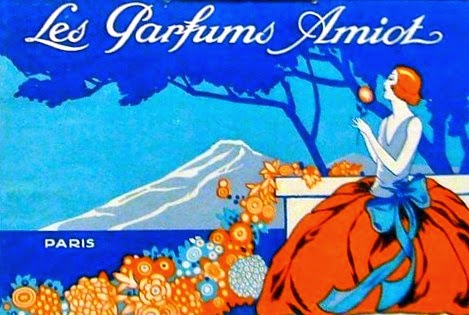This horizontally oriented image appears to be a vintage French advertisement or postcard for perfume, featuring the elegant title "Les Parfums Amiot" in cursive white font outlined in black at the top. The background depicts a serene scene with a cerulean blue sky, a light bluish-gray mountain, and a blue silhouette of a tree. The bottom left corner of the image bears the word "Paris" also in a white cursive type.

In the composition, a woman with fair skin and striking red hair is prominently featured. She is dressed in a blue sleeveless V-neck top and a voluminous red skirt with a large blue bow. The woman is depicted holding and smelling an orange flower, her gaze directed towards the left. She stands amidst a cascading garland of orange and teal flowers that flows from an invisible platform behind her down into a body of blue water. This artistic representation captures a moment of delicate interaction with nature, underscored by the mountainous landscape in the background.